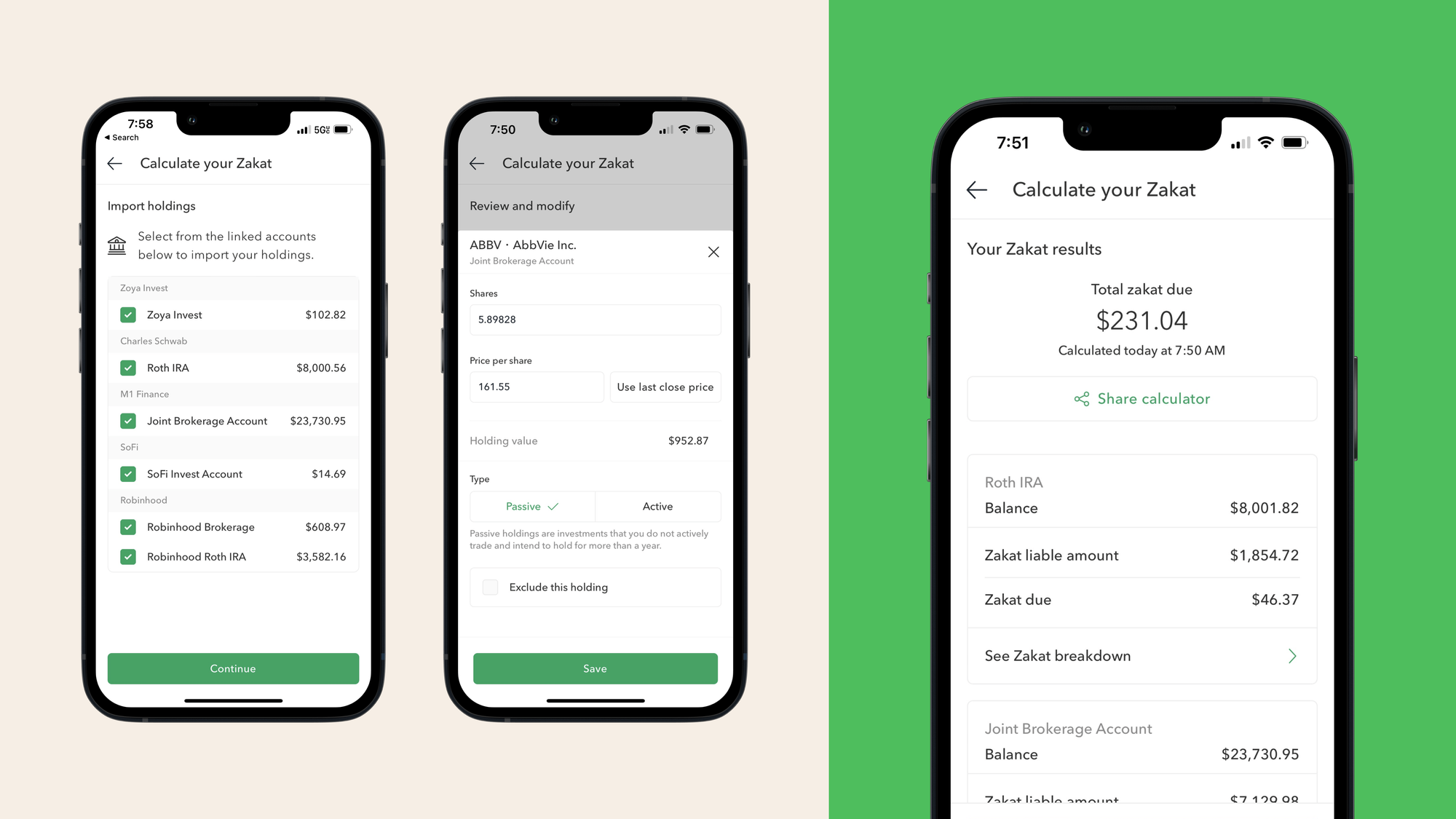This is a detailed caption for the image:

The image showcases a triptych screenshot from a Zakat calculation app displayed on a mobile phone. The layout includes three separate phone screens: two positioned side by side and a third, enlarged, on the right against a vivid green background, detailing the results of the Zakat calculation.

The first phone screen, located on the left, displays the "Import Holdings" menu. Below the menu title, the instructions read, "Select from linked accounts below to import your holdings." The screen lists six financial institutions in a left column, each associated with specific amounts displayed in the corresponding right column.

The middle phone screen presents the "Review and Modify" menu. Beneath this heading, it lists "ABBV-ABBVIENC Joint Brokerage Account", followed by the share details which are somewhat small and difficult to discern: shares at 5.89829, a price per share of $161.55, and an actionable button labeled "Use Last Close Price." The holding value is presented as $9.5287.

Lastly, the enlarged phone screen on the right prominently features the Zakat results. At the top, it reads "Your Zakat Results," and below, the total Zakat due is calculated as $231.04. Additionally, a timestamp indicates that this calculation was completed today at 7:50 AM.